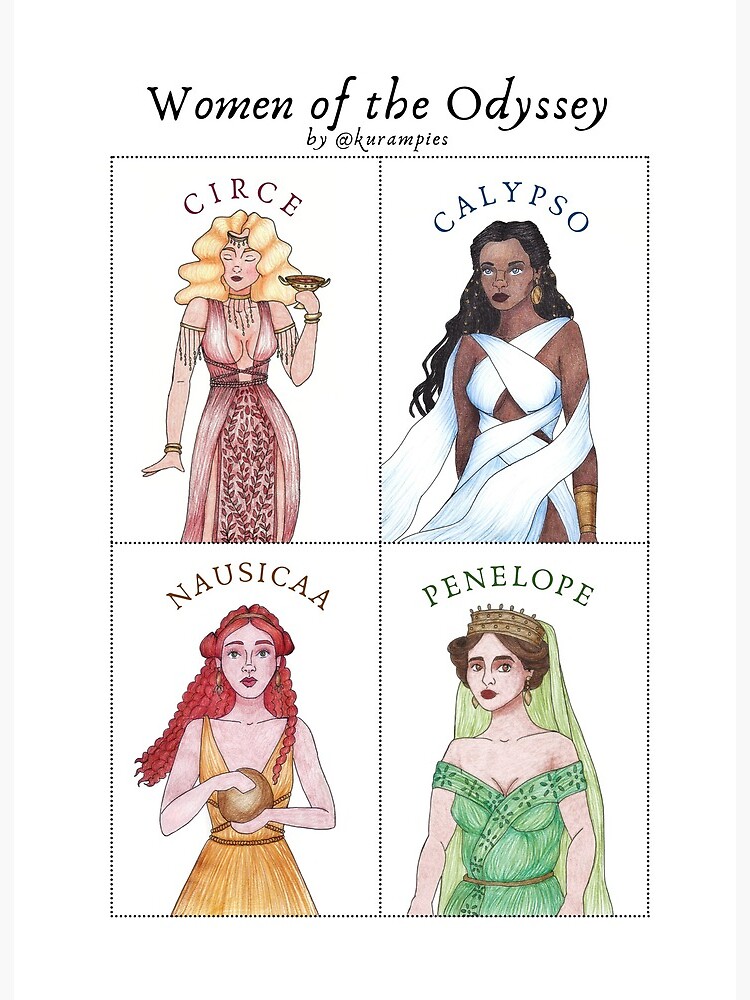The image titled "Women of the Odyssey by Ats Kurampais" showcases four framed artworks of women from the Odyssey. Each woman is depicted with distinct features and attire. From top left, Circe is shown wearing a provocative red dress, holding a cup, and has long blonde curly hair. Next to her, Calypso, a dark-skinned woman with long dark hair, is adorned in a white dress with varying widths, leaving a lot of skin exposed, and she bears an angry expression. Below them, on the left, Nausicaa has red hair and is dressed in a gold-strapped yellow gown while holding a gold orb. Finally, to the bottom right, Penelope, with brown hair and wearing a crown, is elegantly dressed in a green gown. Each character's attire and expressions highlight their unique personas and roles in the Odyssey.